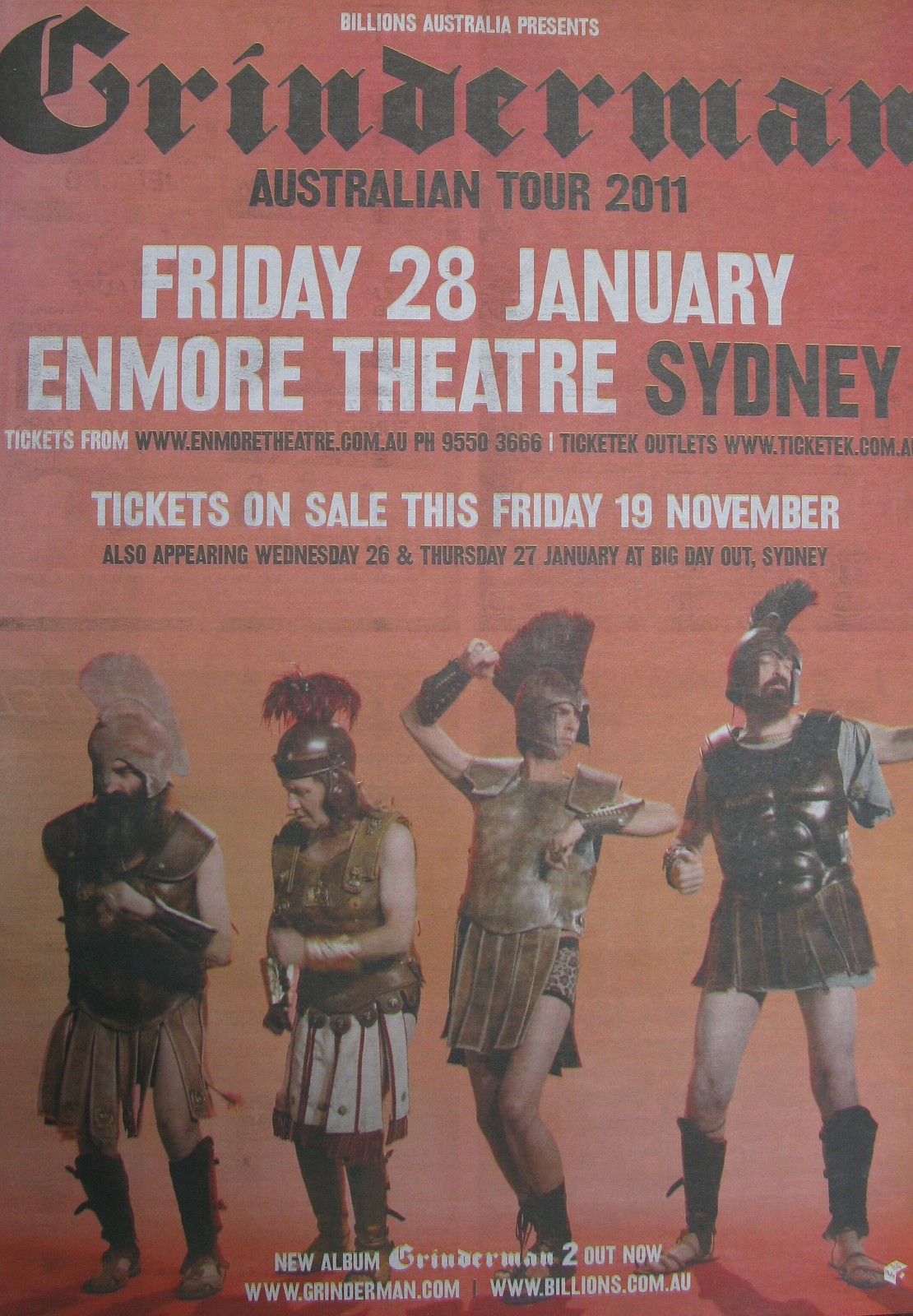The image is a detailed poster for the Grinderman Australian Tour 2011, presented by Billions Australia. It has a red rose-colored background that fades to a lighter shade towards the bottom. At the top, in small white letters, it reads, "Billions Australia Presents," followed by the large black text, "Grinderman" in a medieval-style font. Below this, in smaller black letters, it announces "Australian Tour 2011." The key event details are prominently displayed in large white font: "Friday, 28th January, Enmore Theatre, Sydney." Additional ticket information is included, stating that tickets can be purchased from www.enmoretheatre.com.au and www.tickettext.com.au, with the phone number PH 9550-3666 for ticket inquiries. It also mentions that tickets go on sale on Friday, 19th November, and that Grinderman will also appear on Wednesday, 26th, and Thursday, 27th January, at Big Day Out, Sydney.

The lower half of the poster features four men dressed in light combat gear reminiscent of Roman soldiers. They wear Trojan-style helmets with Mohawk crests, metal vests, short leather skirts, and strap boots, and they are shown in various poses. The predominant colors in the image include red, black, white, gray, brown, maroon, tan, silver, gold, and bronze, creating a visually striking and detailed promotional poster.